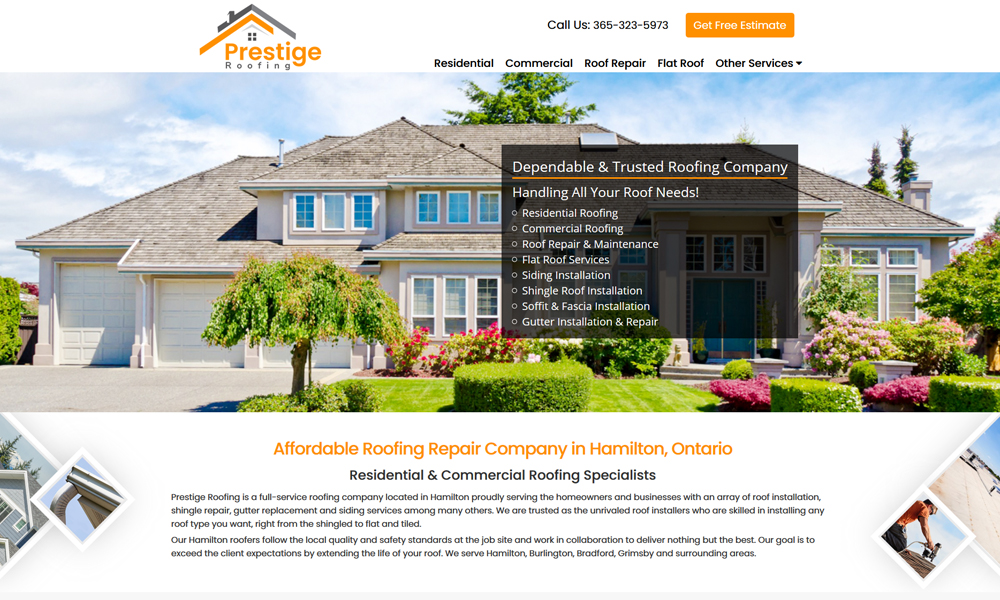The advertisement, titled "Prestige Roofing," features a prominent logo on the top left corner. The logo consists of the word "Prestige" in orange and "Roofing" in black, with an icon of two roofs above: a grey roof on top and an orange roof below, accompanied by four black windows. On the top right of the advert, an orange banner announces "Get a free estimate," with a contact number, 365-323-5973, positioned just to the left.

At the bottom of the advert, there are tabs labeled "Residential," "Commercial," "Roof Repair," "Flat Roof," and "Other Services," each written in brown on a white background. The center section features a block of white text on a transparent black background, detailing the company’s offerings: "Dependable and trusted roofing company, handling all your roofing needs. Residential roofing, commercial roofing, roof repairs and maintenance, flat roof services, siding installation, shingle roof installation, soffit and fascia installation, gutter installation and repair."

The background of the advertisement is an image of a slightly brown house with a grey roof, adorned with various flowers including crane plants and pink and dark pink flowers. At the bottom, orange text proclaims "Affordable roofing repair company in Hamilton, Ontario," followed by black text that states "Residential and Commercial Roofing Specialist."

A final paragraph describes Prestige Roofing as a full-service company based in Hamilton, serving homeowners and businesses with a comprehensive list of services including roof installation, shingle roof repair, gutter replacement, and siding services. The company is reputed for its skilled installation of various roof types, dedication to quality and safety standards, and commitment to exceeding client expectations. Prestige Roofing serves Hamilton, Ballantyne, Bradford, Grimsby, and surrounding areas.